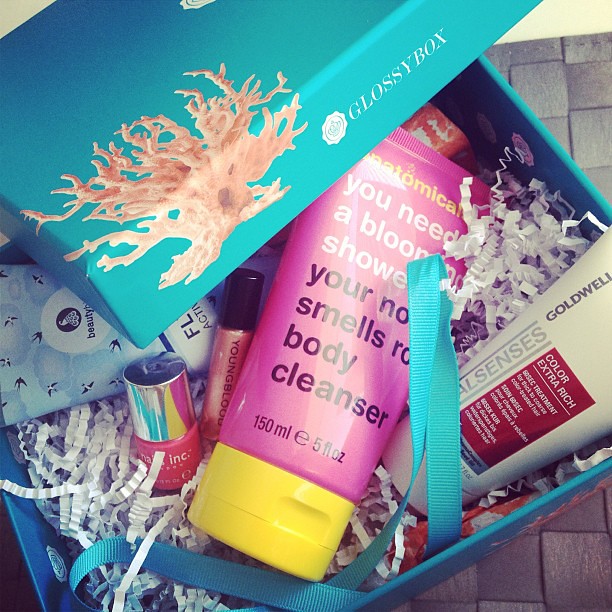This color photograph captures an open aqua-colored Glossy Box, adorned with white text and a salmon-colored coral design on its side. The box, resting on a gray tiled floor, is filled with women's beauty products nestled in shredded packaging paper. Among the visible items is a pink bottle of nail polish featuring a silver top and white text, positioned on the left. Centrally, there's a pink tube labeled "You're No Smells Body Cleanser" in black text, with a yellow cap. Adjacent to it, likely lipstick, is another pink item with a black top that says “Young Blood.” There’s also a white tube labeled "color extra rich," though the smaller text is unreadable. A glimpse of a blue packet is visible among the assortment of toiletries, indicating a diverse compilation of products in the box.